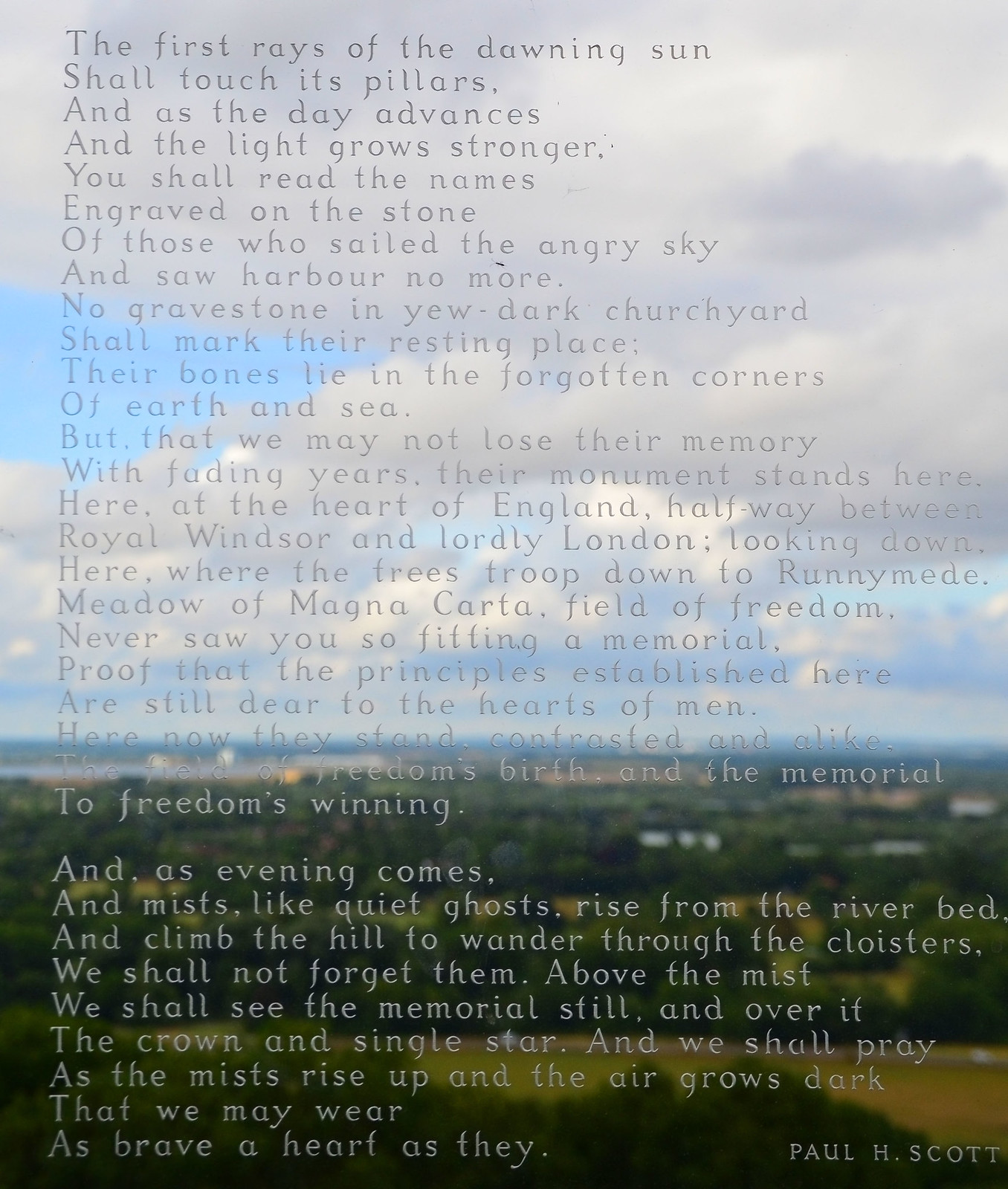In this photograph, we see a poignant poem by Paul H. Scott, his name subtly reflected in the bottom right corner of the image. The poem is overlaid on a serene view of a valley, featuring blue skies interspersed with clouds, lush greenery, and hints of buildings in the background. The text of the poem begins with: "The first rays of the dawning sun shall touch its pillars, and as the day advances and the light grows stronger, you shall read the names engraved on the stone of those who sailed the angry sky and saw harbor no more. No gravestone in you dark churchyards shall mark their resting place. Their bones lie in the forgotten corners of earth and sea, but that we may not lose their memory with fading years, their monument stands here, here at the heart of England, halfway between royal Windsor and lordly land London, looking down here where the trees troop down to Runnymede, meadow of Magna Carta, field of freedom." Although the text is difficult to read due to the light background, the poem invokes a deep reverence, urging that we remember the fallen with fitting memorials, reflecting on the principles of freedom established at this historic field. As evening descends and mists rise from the riverbed to climb the hill, the poem assures us that the memorial will remain visible above the mist, a testament to enduring bravery.